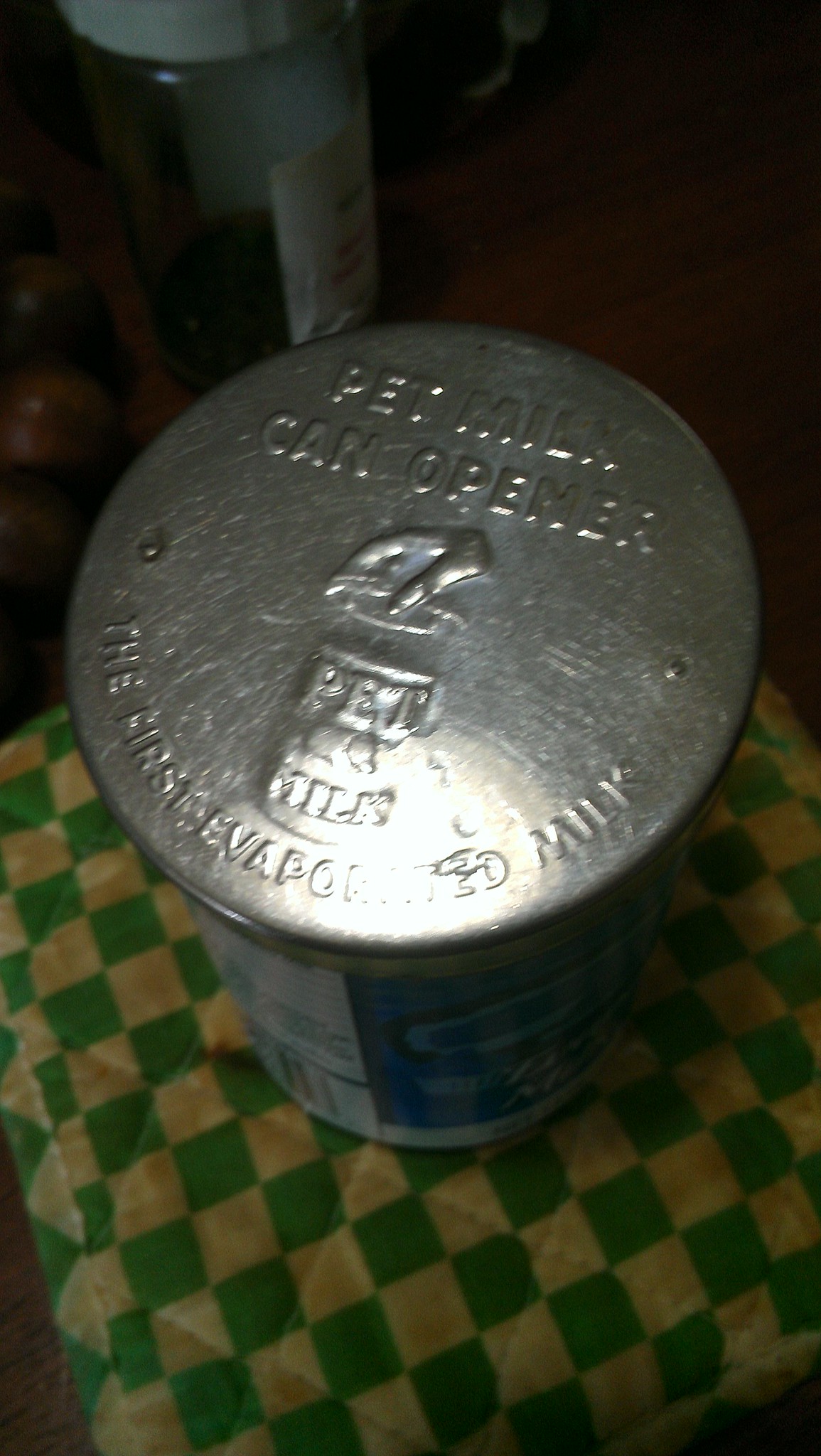In the image, there is an old, silver-topped can prominently labeled "Pet Milk Can Opener - The First Evaporated Milk." This can, which may be a historic or replica example of the first commercially produced evaporated milk, is placed atop a worn, dirty cloth. The cloth has a checkered pattern that appears to have originally been white and green, but age and dirt have left it looking yellow and green. Behind the can, there is a bottle with a label, possibly indicating it contains medication. To the left of the can, there is a lime or some similar fruit adding a touch of color to the scene. The overall setup gives a nostalgic and slightly rustic impression, hinting at a bygone era.